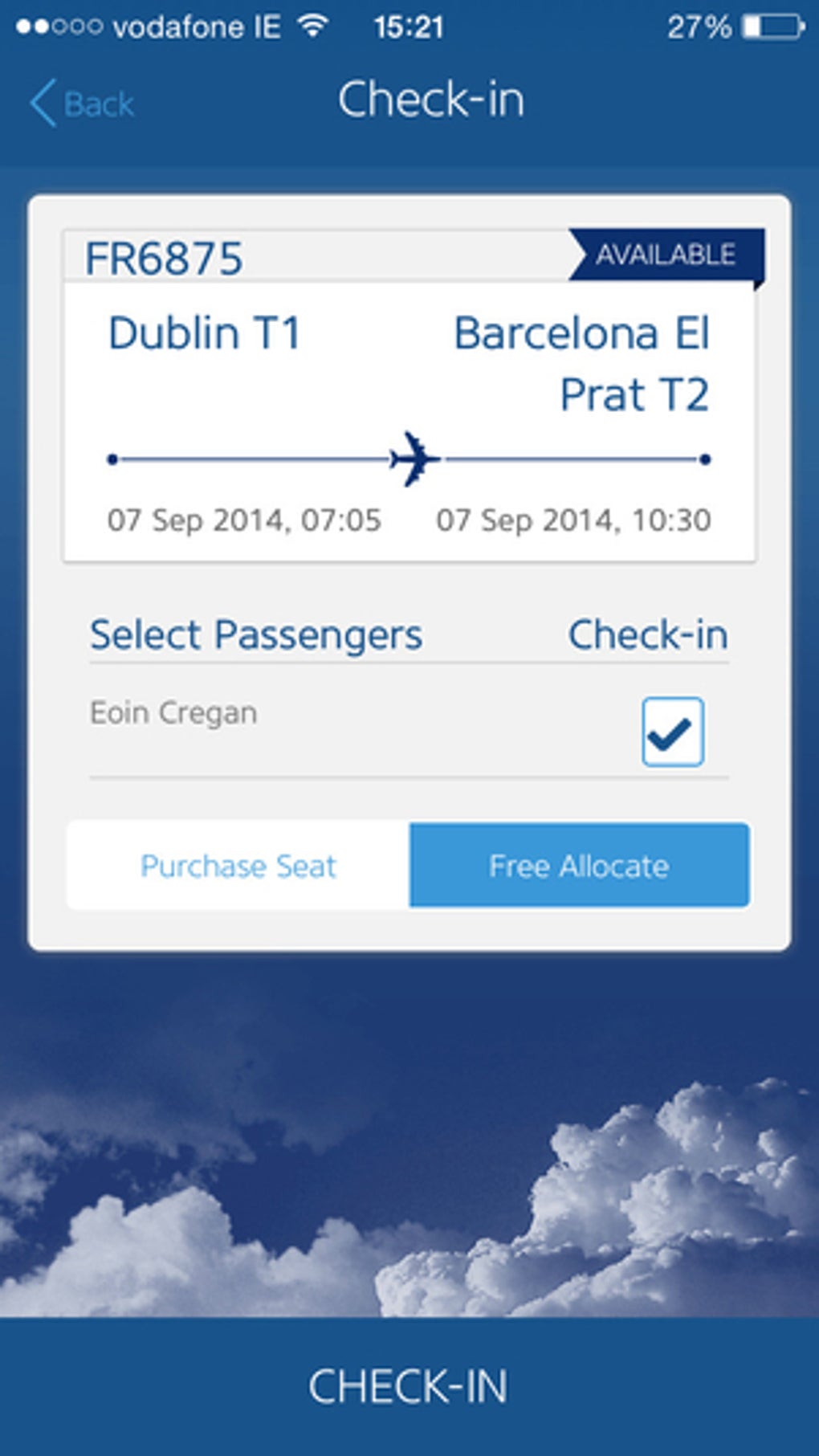The screen capture features a smartphone display, with the provider listed as Vodafone (V-O-D-A-F-O-N-E-I-E). The time displayed on the phone is 15:21, and the battery level is at 27% charge. The focus of the screen is an app interface for a flight check-in. The app is showing a flight from Dublin to Barcelona, indicating availability for check-in. Eoin Creagan (E-O-I-N-C-R-E-G-A-N) is identified as the passenger. The app provides two options: "Free allocate" or "Purchase seat". The background wallpaper of the app displays an image of clouds, contributing to a travel-themed design. At the bottom of the screen, there is a prominent button labeled "Check In".